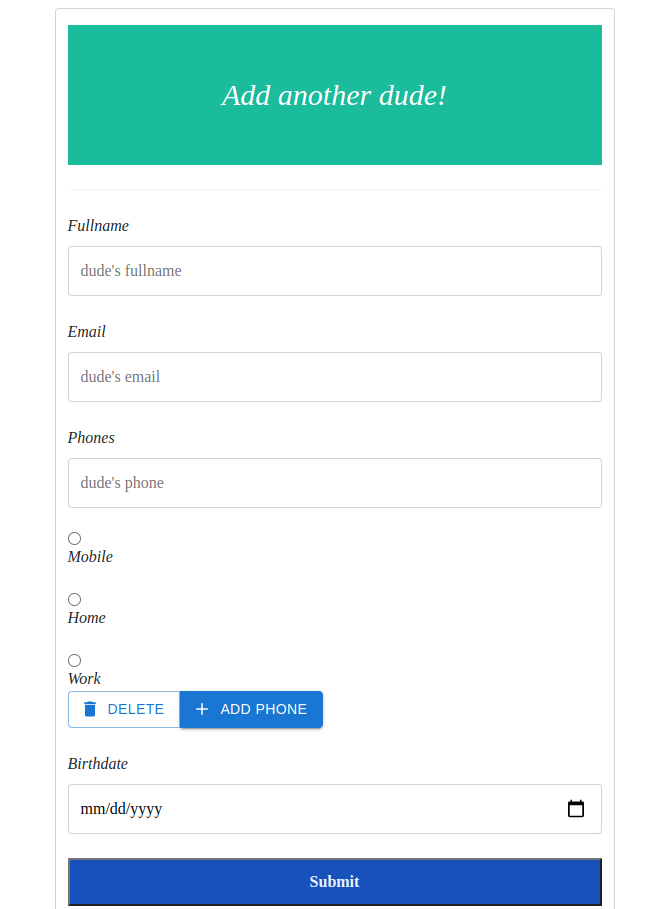Here's a detailed caption based on the provided description:

**Caption:**
A detailed screenshot of an opt-in form characterized by a prominent green header that states "Add Another Dude!" in bold text. The form includes several fields for user information. The first field is labeled "Full Name" with a placeholder text that reads "Dude's full name." Next, the "Email" field shows a placeholder "Dude's email." Following this, the "Phone" field includes a placeholder "Dude's phone." Below the phone number input, there are three radio buttons indicating the type of phone: "Mobile," "Home," and "Work" which can be selected or changed. The form also includes a "Birthdate" field featuring a clickable calendar icon for easy date selection. Toward the end, a prominent blue "Submit" button is located at the bottom of the form, inviting final action on the entry. Each input field is clearly segmented, providing a streamlined and user-friendly layout for data entry.